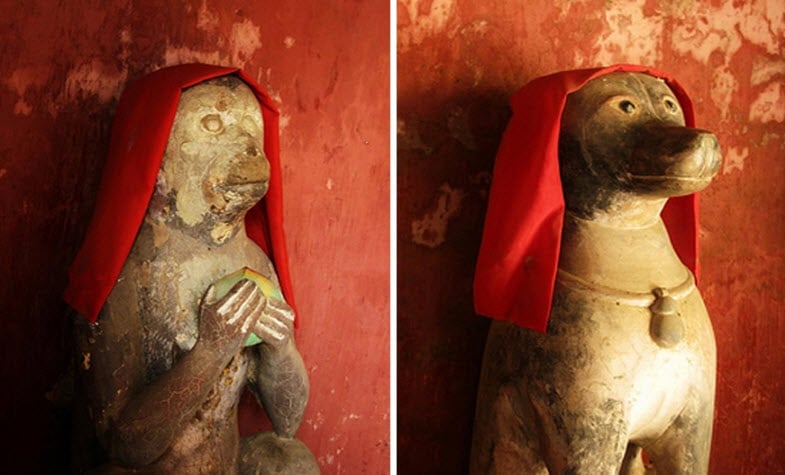The image consists of two photographs, each showcasing a gold patinaed statue set against a distressed red wall with white markings. On the left, there is a monkey statue, holding what appears to be a fruit, possibly greenish in color. The monkey's face is notably worn, and it wears a red cloth draped over its head and shoulders. To the right, a pharaoh dog statue stands, mirroring the red head covering and backdrop. The dog statue, also showing signs of age, features a prominent collar with a large emblem hanging from it. Both statues exude an aged, worn aesthetic, contributing to a coherent and historical ambiance in the scene.